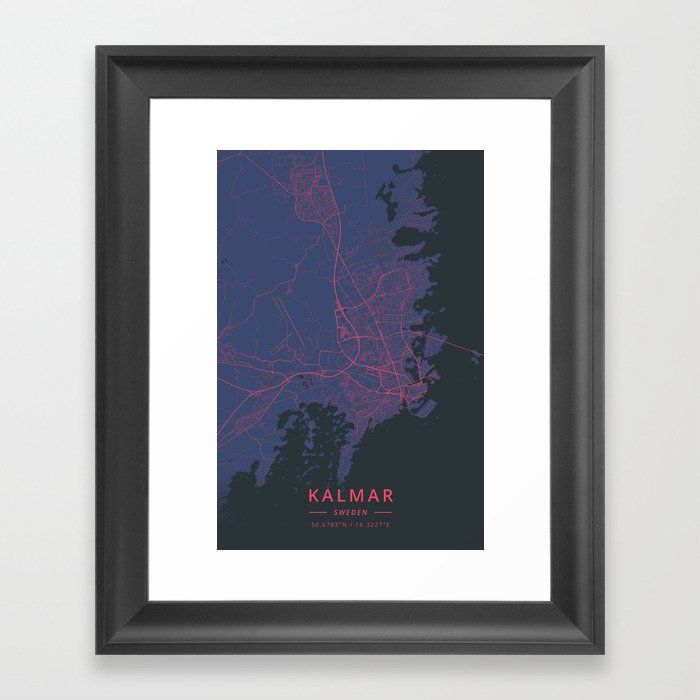The image displays a large, square photograph framed with a simple black border and a broad white mat. The composition features a vertical rectangular picture harmoniously blending hues of blue, pink, and black. The background wall appears light gray but is actually meant to be white. The artwork inside the frame seems to be a stylized map of Kalmar, Sweden. Predominantly, the left portion of the image is a dark navy blue, representing the sky, while pinkish-red lines delineate roads or streets. Black areas illustrate the land with a jagged coast visible at the bottom and along the right side. Below the map, in bold pink all-caps text, is the label "KALMAR." The text "SWEDEN" is flanked by dashes, with an additional set of smaller, barely readable coordinates underneath.